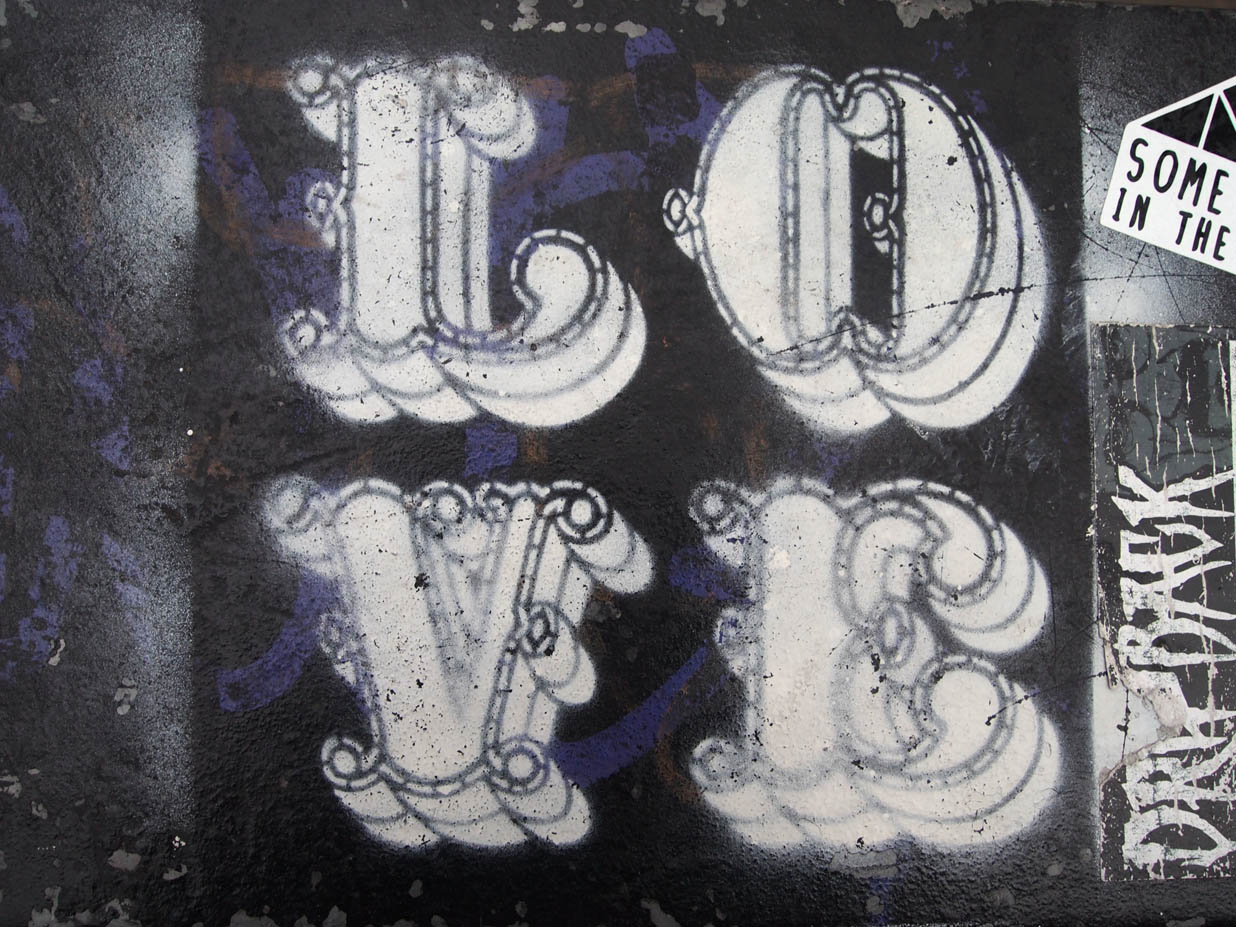The rectangular image depicts a piece of graffiti art against a dark gray wall, which is heavily adorned with various artistic elements. Dominating the center is a meticulously stenciled and ornately designed word "LOVE," arranged in two rows with "L" and "O" on the top row and "V" and "E" on the bottom row. These letters are boldly colored in white with distinctive black outlines, enhancing their visibility against the dark background. The backdrop features predominantly black hues interspersed with vibrant blue and orange lines. On the right side of the image, there is additional graffiti, including a rectangular area with white text that is partially legible, reading "sum in the," along with a vertical, intricate, and somewhat obscured script that seems to spell out "dre bag." The overall scene bears the hallmarks of street art, reflecting a raw, urban aesthetic commonly seen on the sides of buildings or walls, with an eclectic mix of white spray paint splotches adding to the gritty, artistic ambiance.